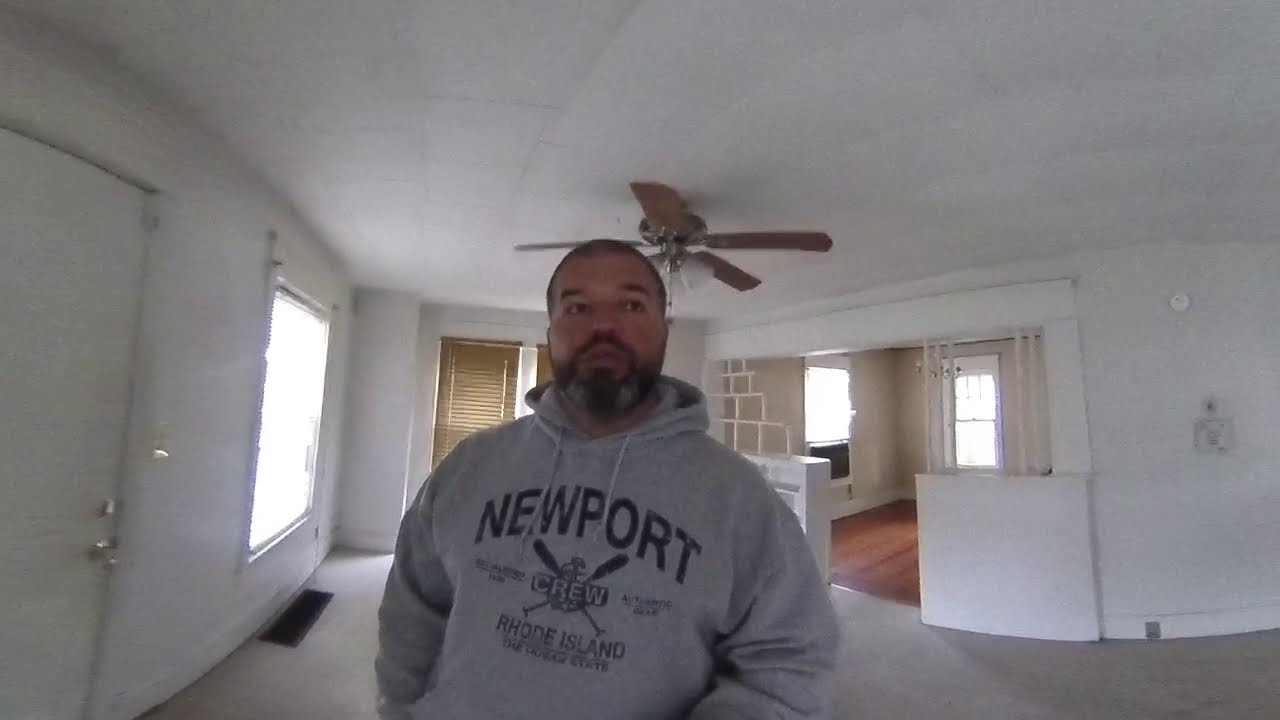A man with short dark hair and a salt-and-pepper beard stands in the middle of an empty living room, wearing a gray hoodie that reads "Newport, Rhode Island, Crew" with a design featuring crossed paddles and an anchor. The living room is characterized by its white walls, white ceiling, and white carpet. To the left of the man, there is a main door and a large square window with sunlight streaming through, casting light over a small black rag on the carpet below. Behind him, brown blinds cover another window, and a brown ceiling fan with two white lights hangs above. Further back, a half wall with an open partition leads into another room with wooden flooring. This adjacent room contains two windows, one on either side of the space. In the room with the wooden floor, a window unit is installed in one of the windows, enhancing the sense of an unoccupied and perhaps recently inspected home.